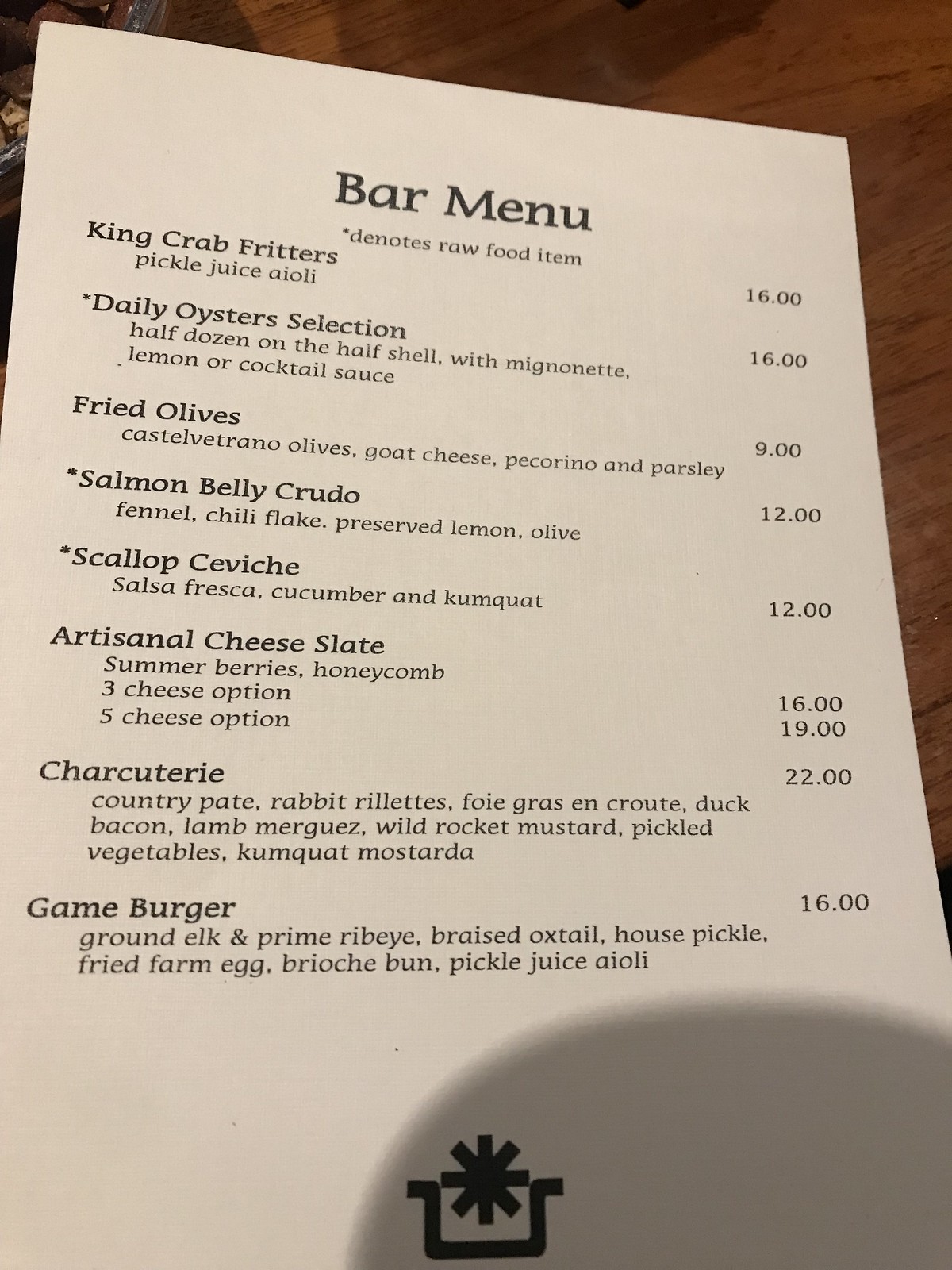The image showcases a detailed paper bar menu on an off-white sheet, resting on a brown dining table. There is a noticeable shadow partially covering the bottom right section of the menu. At the top, the words "Bar Menu" are prominently displayed. 

Underneath, an asterisk notation indicates that specific items denote raw food. 

The menu items include:
- **King Crab Fritters** with pickle juice aioli, priced at $16.
- **Daily Oyster Selection** featuring a half dozen oysters served with mignonette lemon or cocktail sauce, priced at $16.
- **Fried Olives** which are Castelventrano olives stuffed with goat cheese, pecorino, and parsley, priced at $9.
- **Salmon Belly Crudo** (denotes raw food item), prepared with fennel, chili flake, preserved lemon, and olive, priced at $12.
- **Scallop Ceviche** (denotes raw food item), served with salsa fresca, cucumber, and kumquat.
- **Artisanal Cheese Slate** accompanied by summer berries and honeycomb, available in a three cheese option for $16 or a five cheese option for $19.
- **Charcuterie Selection** includes country pate, rabbit rillettes, foie gras en croûte, duck bacon, lamb, wild rocket mustard, pickled vegetables, and kumquat mostarda, priced at $22.
- **Game Burger** featuring ground elk and prime rib eye, braised oxtail, house pickle, fried farm egg, brioche bun, and pickle juice aioli, priced at $16.

The menu items are meticulously detailed, showcasing a range of gourmet dishes that blend unique ingredients and flavors.